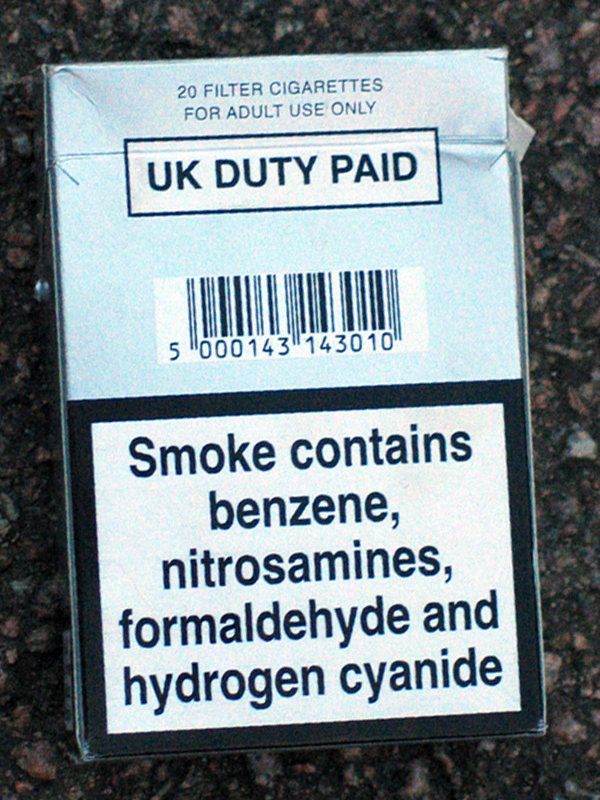This image is a close-up of the back of a cigarette box, resting on a dark, black and white marble or granite countertop. The box is primarily silver in color with distinct black and white text. At the top, it reads "UK duty paid" and "20 filter cigarettes for adult use only." Beneath this, there is a barcode on a small white background. The bottom half of the cigarette box has a narrow black frame, enclosing a white background with large, bold black text that warns, "Smoke contains benzene, nitrosamines, formaldehyde, and hydrogen cyanide." The shot is tightly cropped, showing no people or additional objects.